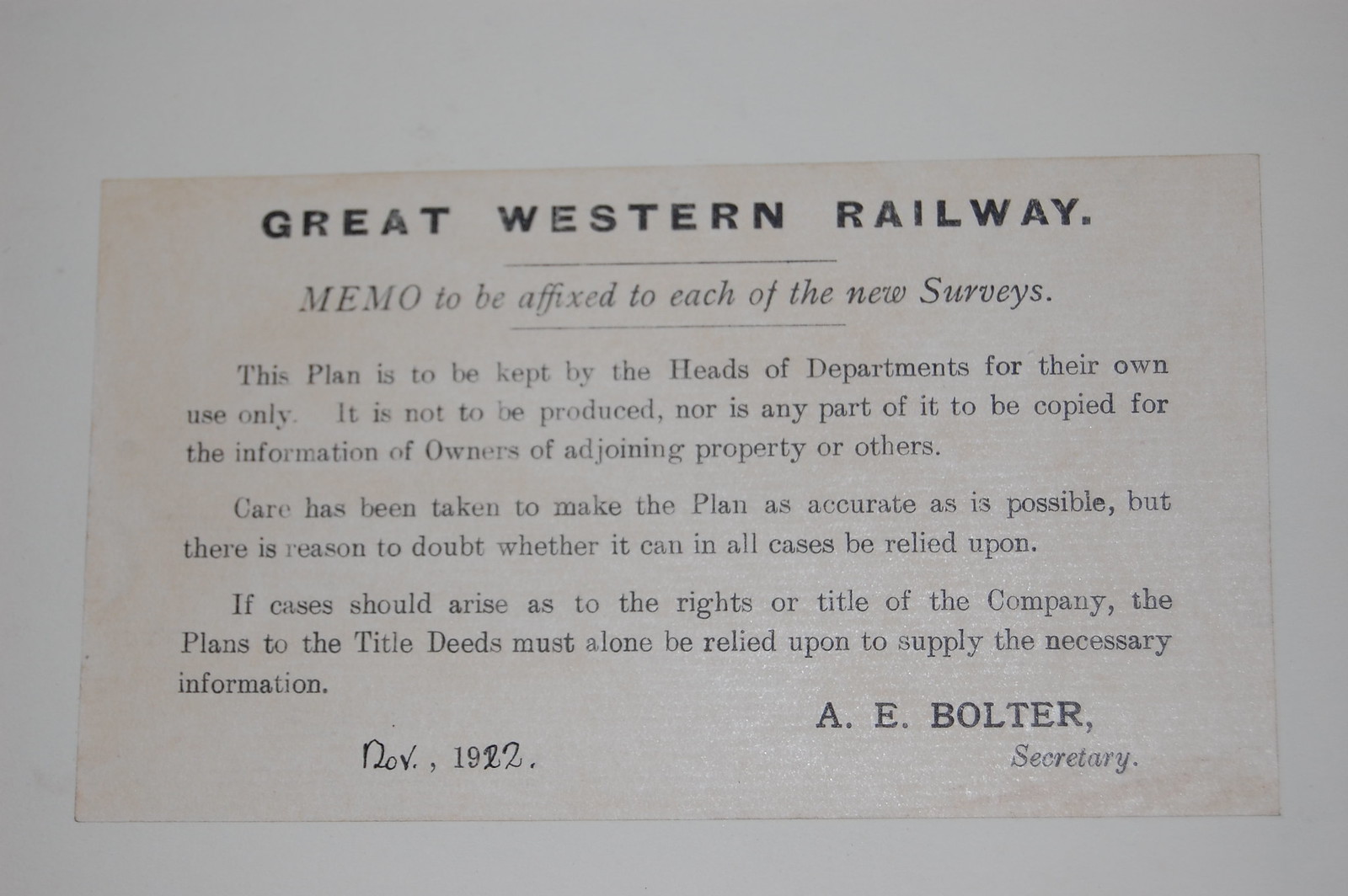The image captures a single rectangular memo placed on a clean, solid white surface, drawing focus directly to the aged document in the center. The memo, printed on a once-white but now yellowed paper due to age, prominently features the heading "Great Western Railway" in bold at the top. The printed black text beneath includes the instruction, "Memo to be affixed to each of the new surveys. This plan is to be kept by the heads of departments for their own use only. It is not to be produced nor is any part of it to be copied for the information of owners of adjoining property or others. Care has been taken to make the plan as accurate as possible, but there is reason to doubt whether it can in all cases be relied upon. If cases should arise as to the rights or title of the company, the plans to the title deeds must alone be relied upon to supply the necessary information." This historically significant document is dated November 1922 and signed by A. E. Bolter, Secretary. Its practical yet cautionary content reflects its purpose within Great Western Railway's operational directives, emphasizing the exclusivity and tentative accuracy of the plans mentioned.